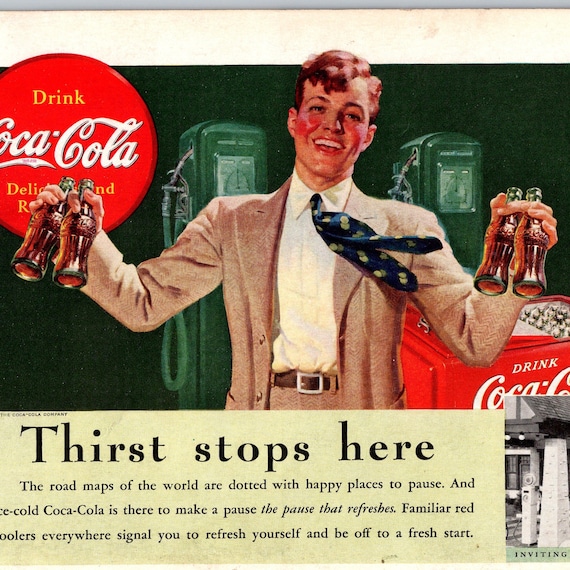The advertisement features a vintage image of a young man with brown hair and rosy, painted cheeks, dressed in an old-fashioned beige suit, a light yellow shirt, and a navy blue tie with yellow polka dots. He stands with a cheerful expression, holding two Coca-Cola bottles in each hand. Behind him, a retro gas station scene unfolds, complete with fuel pumps and red Coca-Cola coolers. A distinctive Coca-Cola vending machine is also visible. The advertisement has a gray border at the top, transitioning into a light pink background. Prominently placed in the top left corner is the iconic red Coca-Cola logo with the words "Drink Coca-Cola." At the bottom left, text reads: "Thirst Stops Here. The roadmaps of the world are dotted with happy places to pause. An ice-cold Coca-Cola is there to make a pause, the pause that refreshes. Familiar red coolers everywhere signal you to refresh yourself and be off to a fresh start."